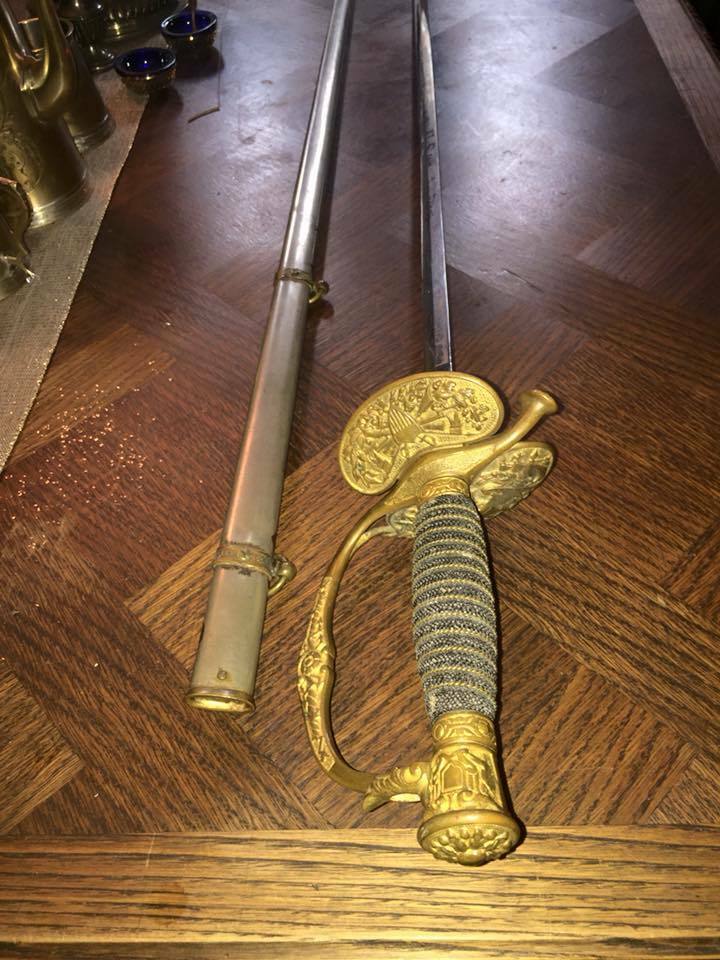In the photograph, we see a meticulously detailed, antique officer's saber, possibly a ceremonial captain's saber from the 1700s or 1800s, prominently displayed on an ornate wooden tabletop, which resembles mahogany. The shot captures the saber and its accompanying scabbard, both exuding a sense of historical significance and craftsmanship. The saber’s handle features a tightly wound fabric grip adorned with a gold-plated handguard that includes an image of a shield with stripes at the bottom and a solid top, suggesting an American military origin. The blade is short, narrow, and straight, potentially hinting at its ceremonial purpose. The scabbard, lying parallel to the saber, has a silver-bronze hue with gold loops at intervals, enhancing its elaborate appearance. Surrounding the saber, partially visible, are various metal bowls and pots, adding to the historical ambiance. The scene is lit by both natural light from an off-camera window and a camera flash, which accentuates the gold elements of the saber’s hilt.